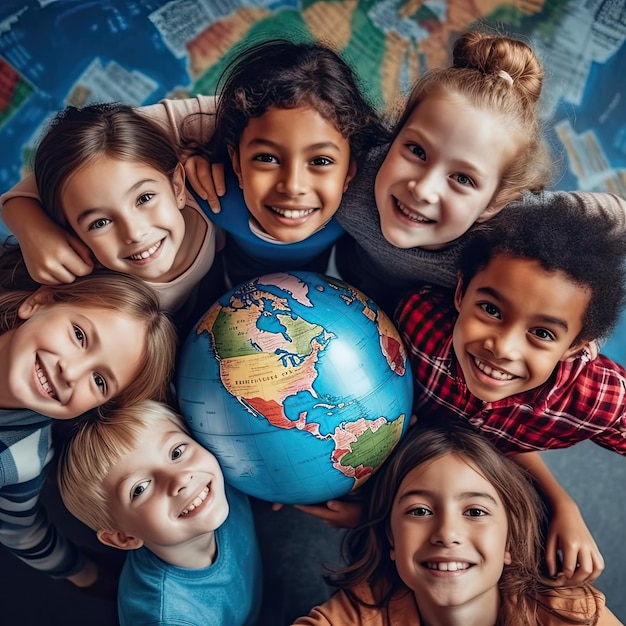In this captivating aerial photograph, a circle of seven smiling children is captured, eagerly looking up at the camera. At the center of their formation rests a detailed globe, tilted to prominently display the United States. The scene is set against a vivid floor patterned in blue, green, brown, and white, mimicking the oceans and diverse terrains of the world. The children, arranged around the globe, include a little girl with brown hair, a boy with black hair, a girl with blonde hair, a girl with dark hair and darker skin, a girl with brown hair wearing a brown shirt, another girl with blonde hair, and a boy with light blonde hair donning a red flannel shirt. Their infectious smiles, their diverse appearances, and their close formation suggest a joyful unity and curiosity about the world they are gathered around.